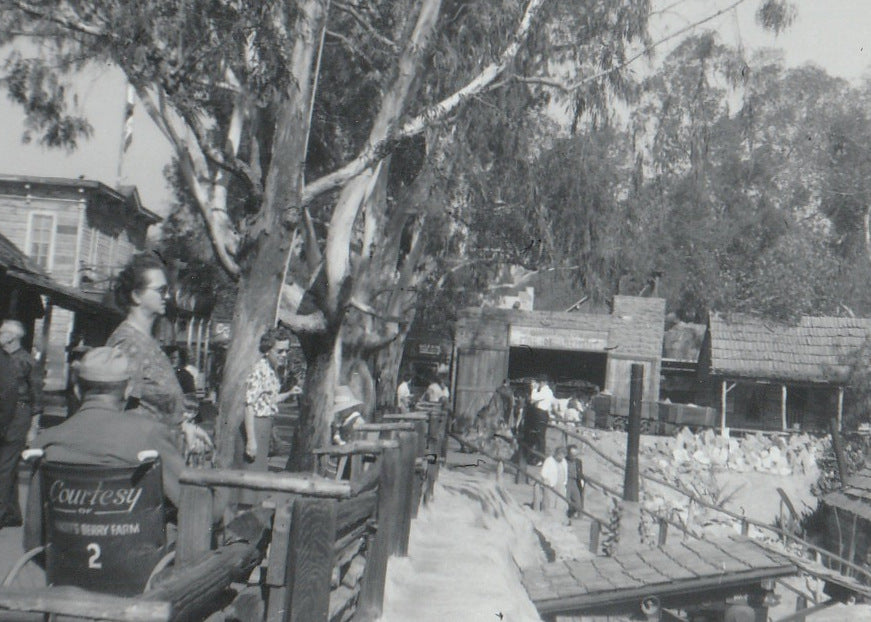The black and white photograph depicts an old western-style scene featuring approximately ten people, all seemingly older, spread across the image and facing various directions. In the foreground, on the left side, there is an older woman wearing sunglasses looking to the right, while behind her sits a man in a wheelchair labeled "Courtesy of Knott's Berry Farm" with "number 2" at the bottom. The scene includes wooden buildings and a line of trees in the background, contributing to its vintage feel. The setting appears to be an open area, possibly a pen for livestock, bordered by a wooden fence. To the left, there is some visible vegetation, and the overall image has a slightly blurry quality. The photograph captures a mix of people, buildings, and natural elements in a moment reminiscent of a bygone era.